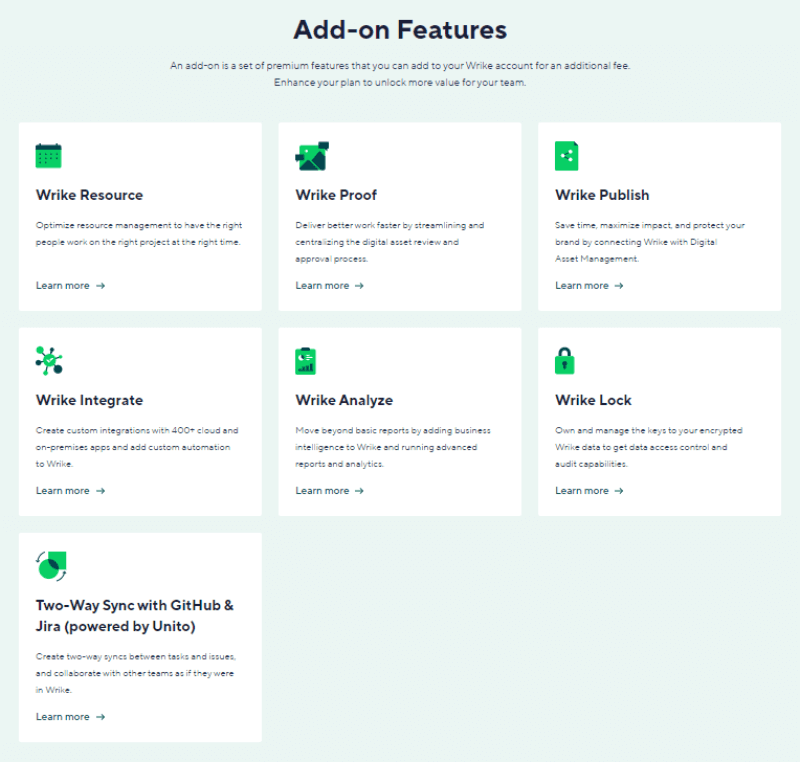The control panel of a website displays a very light green background with black text. It features seven distinct white square boxes within the body of the webpage. At the very top, a heading reads "Add-On Features," followed by a description: "An add-on is a set of premium features that you can add to your Wrike account for an additional fee. Enhance your plan to unlock more value for your team."

The options for these add-ons are listed as:
- Wrike Resource
- Wrike Proof
- Wrike Publish
- Wrike Integrate
- Wrike Analyze
- Wrike Lock
- Two-way sync with GitHub and Jira powered by UNITO

Wrike, spelled W-R-I-K-E, appears to be the name of the website offering these add-ons. Among the various services listed, only GitHub, a widely-known platform, stands out as familiar.